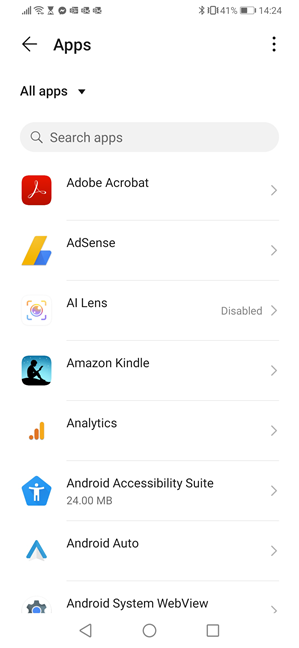The image is a portrait-oriented screenshot of a smartphone screen taken at 14:24 with a 41% battery level, as indicated in the upper right corner. The header features a back arrow on the left and the word "Apps" in bold black text to the right. Below this header, there's a dropdown labeled "All apps" and a gray search bar that says "Search apps".

The main part of the screen displays a vertical list of apps, starting with the letter "A". Each app is represented by its icon on the left and a forward arrow on the right. The list begins with:

1. **Adobe Acrobat** - Icon: Red square with the Adobe logo.
2. **AdSense** - Icon: Yellow and blue logo.
3. **AI Lens** (disabled) - Icon: Camera lens with bordered edges.
4. **Amazon Kindle** - Icon: Blue background with a silhouette of a child reading.
5. **Analytics** (Google Analytics) - Icon: Orange and yellow hues.
6. **Android Accessibility Suite** - Icon not described.
7. **Android Auto** - Icon not described.
8. **Android System WebView** - Icon not described.

The screenshot captures just the beginning of a long list of installed apps, requiring further scrolling or searching to view the rest.